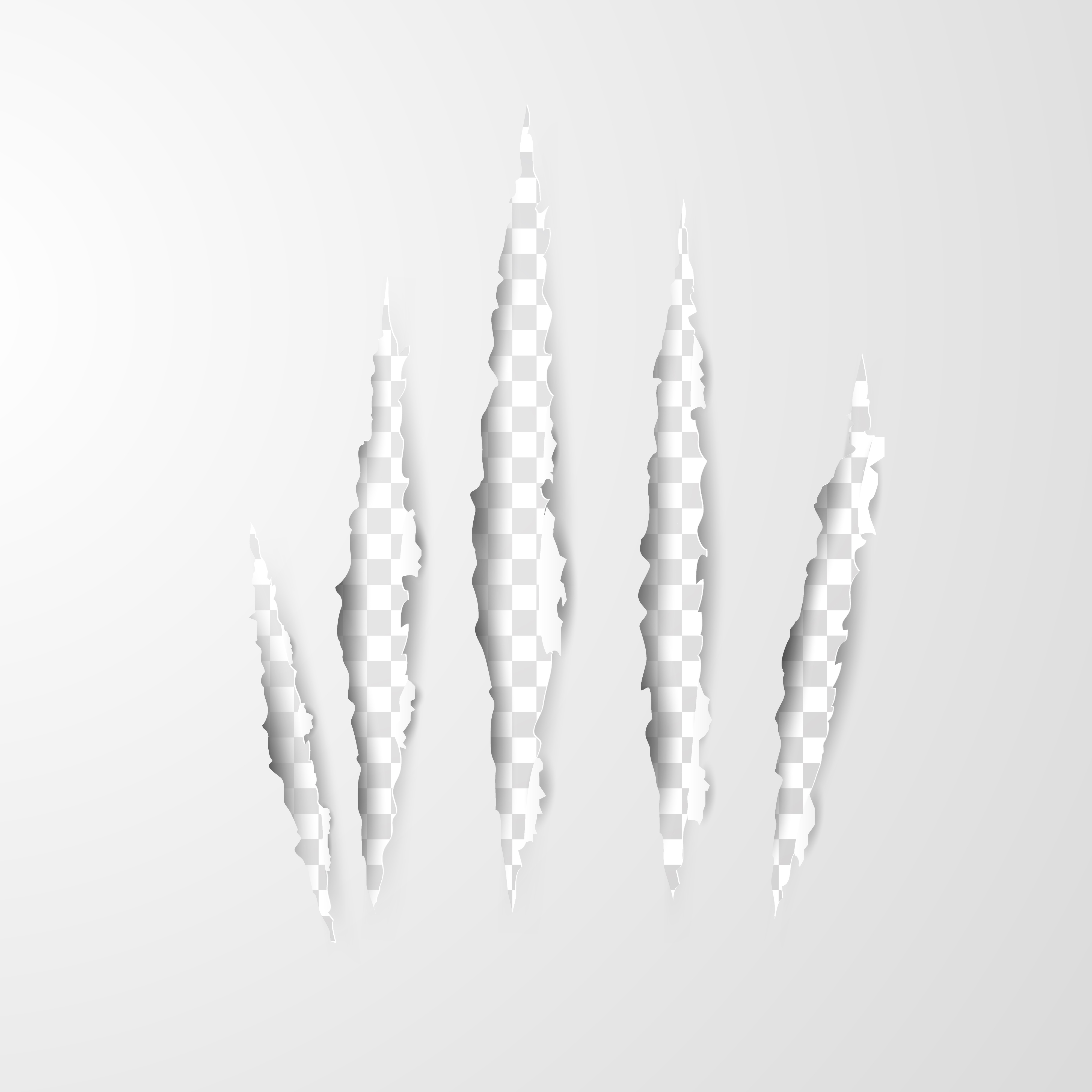This image appears to be a computerized graphic, likely from a graphics e-commerce site, characterized by a square, gradient background. The gradient shifts from a very light gray in the top left to a slightly darker gray at the bottom right. Dominating the center of the image are five vertical tear marks, resembling claw scratches, with jagged edges. These scratches vary in size, with the largest in the center, tapering down towards the edges, indicating a right-hand pattern with the smallest on the left and gradually larger towards the middle before decreasing again. Beneath these tear marks lies a small checkerboard pattern of gray and white, commonly representing transparency in graphic design programs like Photoshop. The overall look is clean, devoid of any text or additional decoration, focusing solely on the detailed depiction of the torn surface and the revealed checkerboard.